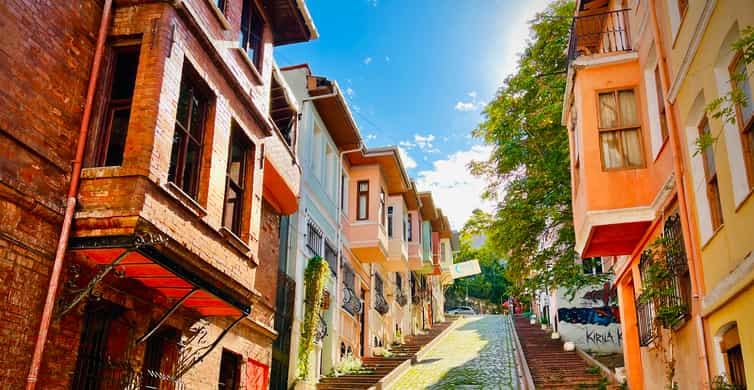This image portrays an AI-generated painting of a quaint, slanted neighborhood, rendered with striking detail. At the center lies a cobblestone walkway, slightly angled upwards, flanked by wooden brown stairs on either side. The walkway, interspersed with green moss, ascends through the heart of this picturesque scene. Lining the left side of the path are a series of closely packed, structurally sound buildings, each distinct in color and character—starting with a red brick building, followed by a blue one, then a pink, an orange, another pink, and finally a blue building further up the hill. On the right, a prominent yellow and orange building overhangs the walkway slightly, featuring a side window and a green tree extending from the overhang. Alongside these buildings, the cobblestone road creates a harmonious blend of old-world charm and architectural sturdiness.

The right side also showcases a white wall adorned with graffiti, featuring blue and red hues and some letters, possibly a “K.” This wall likely encloses a lawn area, adding to the neighborhood's character. Behind these structures, various trees peek through, enhancing the backdrop with natural greenery as the road ascends. Above, the painting is capped with a serene blue sky scattered with fluffy white clouds, casting an idyllic light over this charming sloped street.